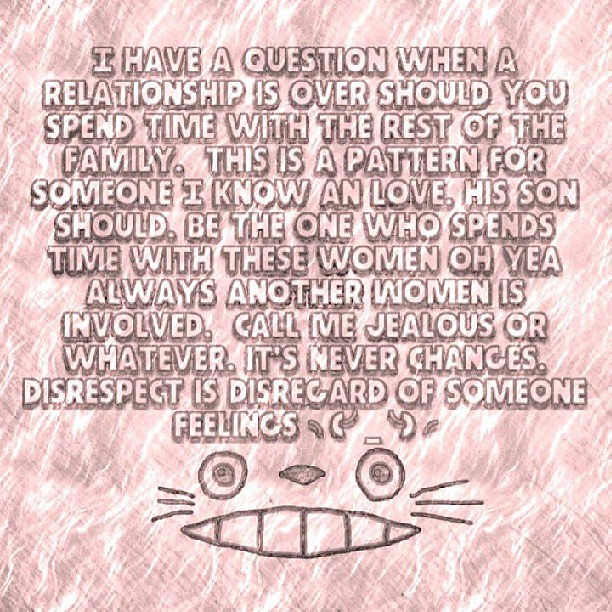This square image features a pink and gray background with text in black block letters, outlined in white. The text, which is written in somewhat broken English, reads: "I have a question. When a relationship is over, should you spend time with the rest of the family? This is a pattern for someone I know and love. His son should be the one who spends time with these women. Oh yeah, always another woman is involved. Call me jealous or whatever. It never changes. Disrespect is disregard of someone's feelings." Below the text, there's a character resembling a Studio Ghibli creation—likely a cat with disconcerted round eyes, a nose, three whiskers on each side, and a toothed mouth—adding to the image's emotional tone. The character and the text together convey a sense of frustration and hurt.